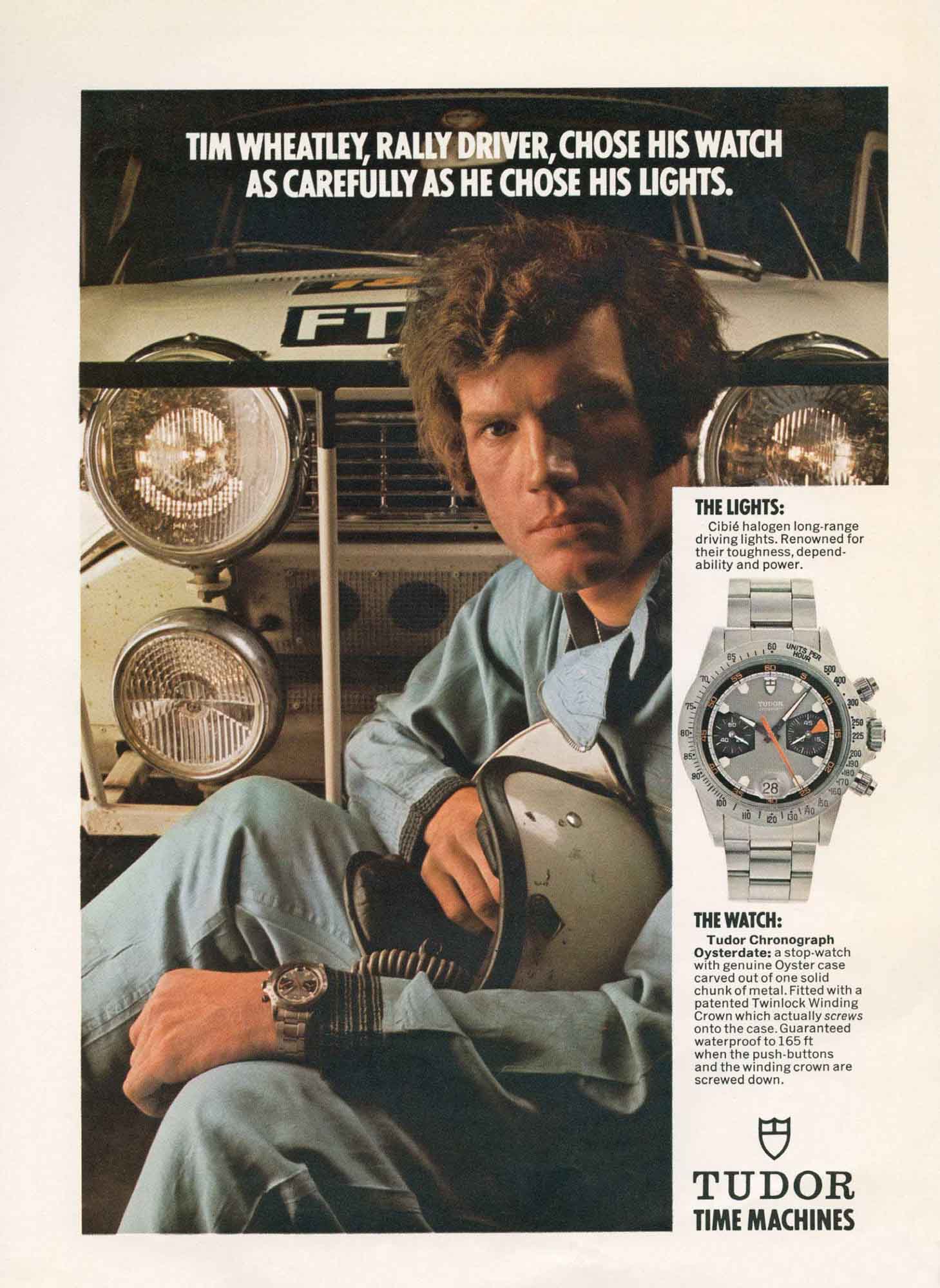The image is a vintage magazine advertisement featuring rally driver Tim Wheatley. Dominating the top center, the text reads: "Tim Wheatley, rally driver, chose his watch as carefully as he chose his lights." The main focus of the ad is Wheatley himself, seated in front of a race car with visible headlights, though part of the text behind him is obscured, suggesting "FT something." He's dressed in a light blue race suit and wears a stern expression, his full lips set in a serious pose. On his wrist, he sports a Tudor watch, and he holds a rally helmet in his hand. The right side of the advertisement showcases the watch, with detailed specifications about its features—including a genuine oyster case, patented twin lock winding crown, and waterproof capabilities up to 150 feet. At the bottom, it proudly declares, "Tudor Time Machines." The overall composition, along with the tagline and detailed features of the watch, reflects a sense of precision and reliability, mirroring the qualities essential in both a rally driver and his equipment.